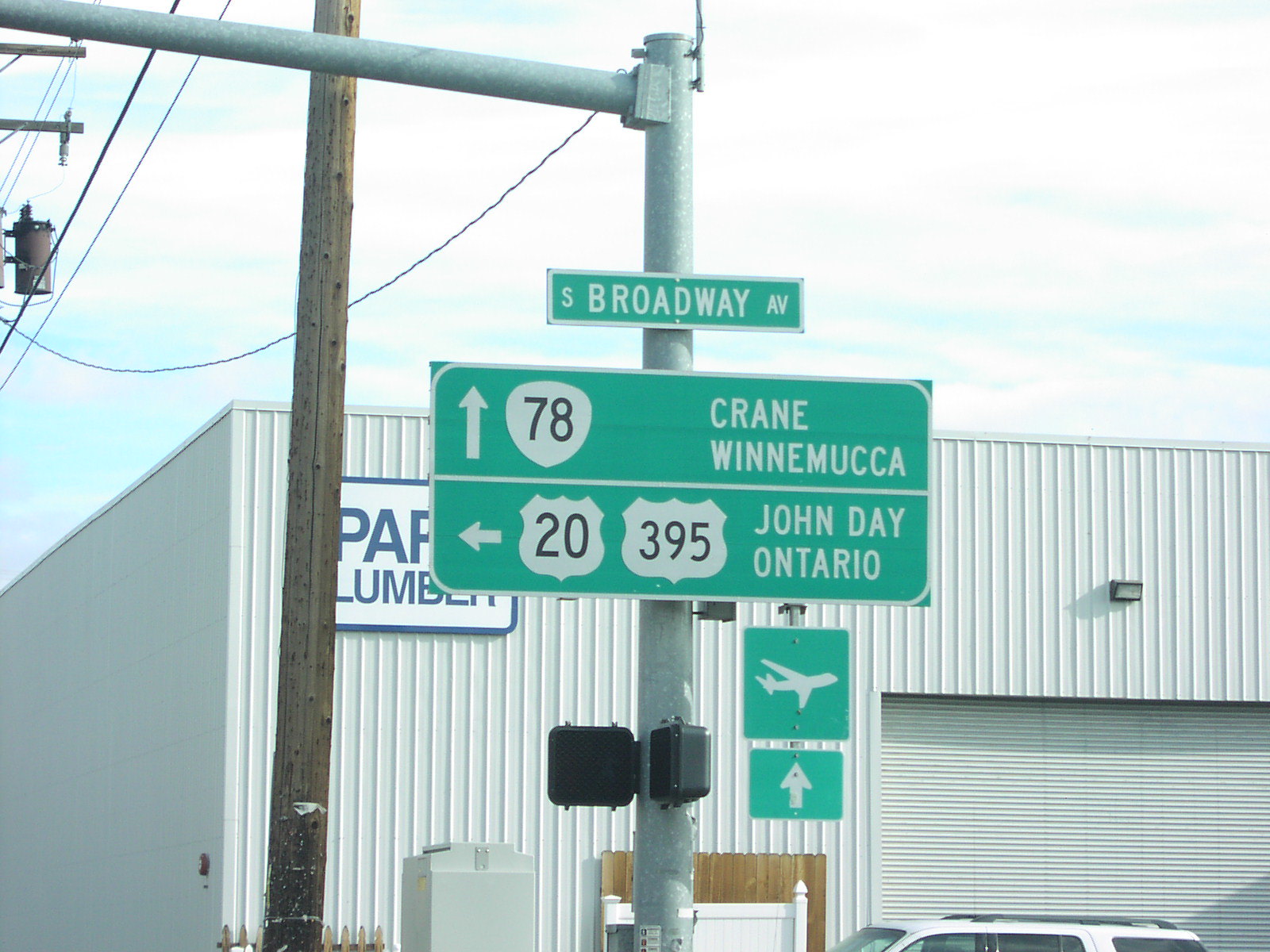This landscape photograph captures street signs at an intersection above a crosswalk. The signs are attached to a pole that also supports a traffic light, which is cropped out of the frame. In the background, a lumber facility is partially visible, with a white building featuring a garage door opening. The facility's name is obscured by the street signs.

The top street sign reads "South Broadway Avenue." Directly below it is an interstate or highway sign for "78," with an upward-pointing arrow and the text "Crane" and "Winnemucca." Another sign beneath shows an arrow pointing left alongside interstate signs for "20" and "395," directing to "John Day" and "Ontario." At the bottom, two symbols indicate the presence of a nearby airport, with an airplane icon and an upward-pointing arrow.